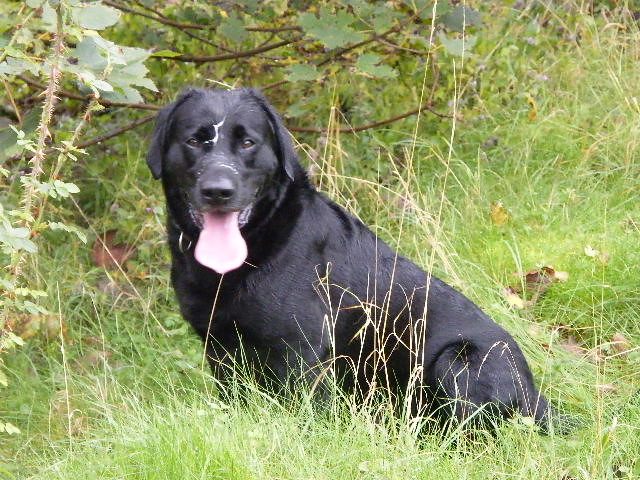The image displays a detailed scene of a full-grown black Labrador with floppy ears, sitting in a grassy field. The dog, distinguished by its entirely black fur and a faint white stripe on its forehead, is looking directly into the camera with its tongue hanging out, indicating it is panting and possibly warm. A collar is visible around its neck, suggesting it belongs to someone. Surrounding the dog is a bed of tall, light green grass, interspersed with loose branches and dead, brown leaves falling to the ground. Nearby, various plants and bushes are visible, with some leaves still green, hinting at a mid-summer or late spring setting. At the side of the dog, a thistle can be seen among the dense vegetation. The Labrador appears sturdy and healthy, adding to its endearing presence in this natural environment.